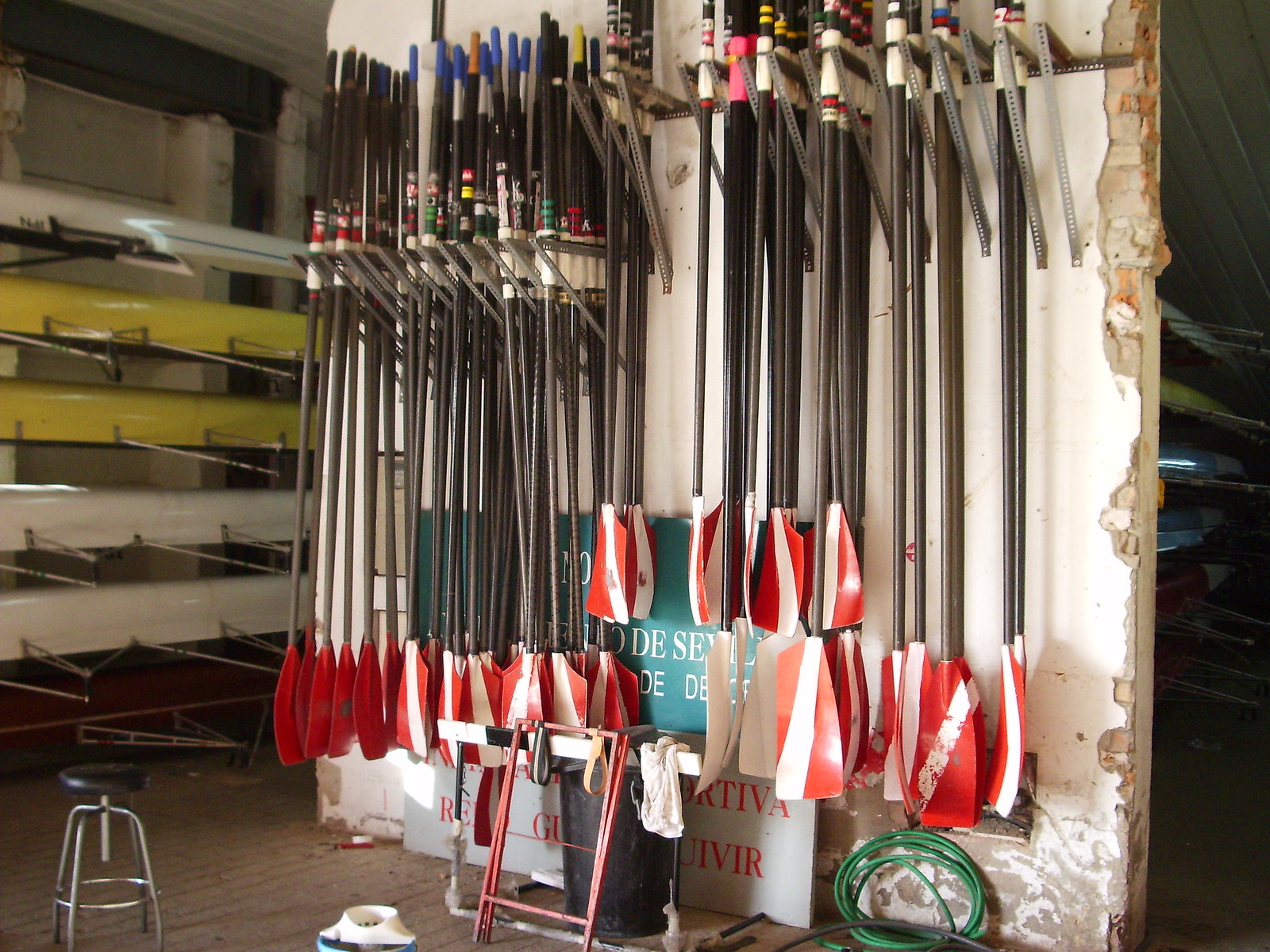This is a square color photograph capturing a section of a wall adorned with approximately 50 paddles, presumably used for paddleboarding or kayaking. These paddles, with assorted elongated handles and differently colored tops, are mounted on five rows of metal brackets secured to a white wall. The bottom edge of the photograph reveals a coiled garden hose to the right and a small red step stool in the foreground. Two Spanish signs are visible on the wall behind the paddles, though they are illegible. The left side of the image shows stacked boats, including two red boats, a blue boat, and a yellow boat, with a small brown stool with grey legs positioned below them. The right edge of the frame fades into darkness, and a small section of the brick wall is visible, exhibiting a break in the plaster.